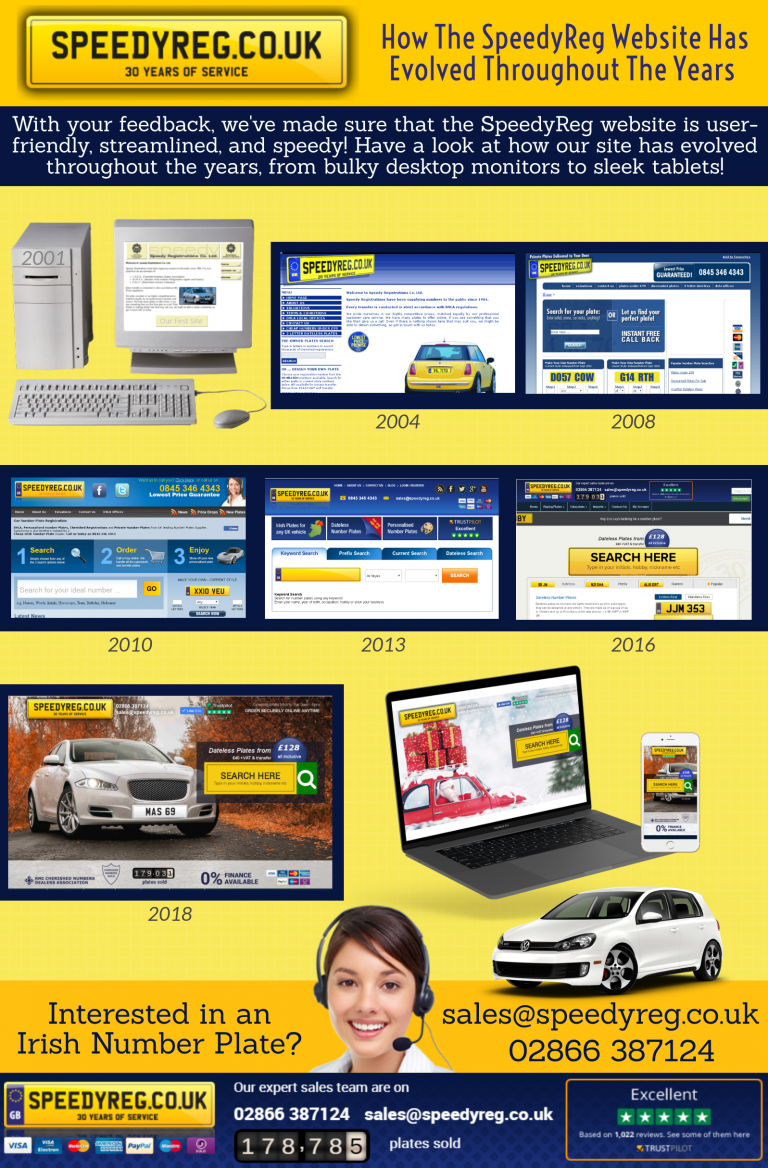This advertisement showcases the evolution of the SpeedyReg website in vibrant yellow and blue colors. In the upper left corner, a bold yellow rectangle features the text "speedyreg.co.uk" in black font, followed by a note celebrating "30 years of service." Adjacent to this, a passage highlights how, with customer feedback, the SpeedyReg website has transformed to become user-friendly, streamlined, and efficient.

Below this text, a timeline of images illustrates the website's progression over the years: starting with an old tower desktop from 2001, transitioning to flat screens in 2004 and 2008, and continuing to more modern flat screens from 2010 to 2018. The final visual showcases the website displayed on both a sleek cell phone and a laptop, representing its current versatility.

Additionally, the advertisement features an image of a white Volkswagen and offers information on acquiring Irish number plates, directing interest to "sales@speedyreg.co.uk" or the phone number "0288-866-387124." A photograph of a young woman with brown hair wearing a white shirt and a headset is also included, emphasizing the availability of sales expert teams at the provided contact details. The ad proudly states, "178,785 plates sold."